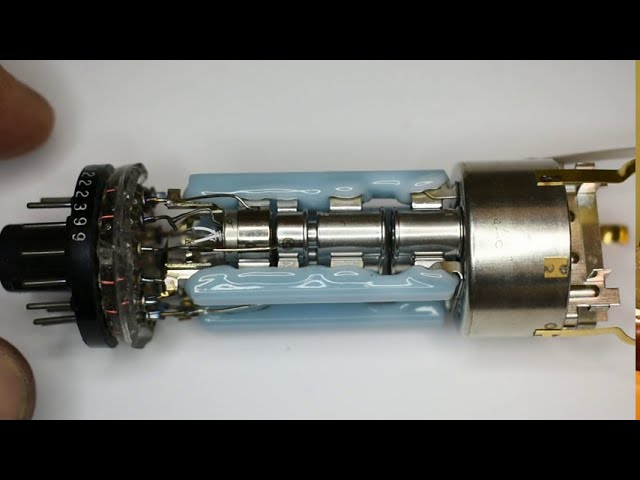The image is a color photograph of a small electrical component, set against a black background with a white piece of paper beneath it. The photograph is framed with thick black borders at the top and bottom, and although not professionally lit, the components are visible. In the left of the frame, you can just see the tips of someone’s forefinger and thumb, indicating the object's small size. The component lies horizontally, from left to right, at the center of the image.

On the left side of the component, there is a black round disk base with white numbers inscribed on it, including "22399." Protruding from this base are numerous slender steel pins encircling a base that plugs into a board. Above the base, the pins progress into an assembly of copper wiring and four barrel-shaped stainless steel sections. These sections have wires running across them, possibly indicating battery cells. A shiny metallic rod runs horizontally through the center of the tube, with light reflecting off its stainless steel surface.

Sealing the top and bottom are thin lateral lines of what appears to be melted light blue plastic. The entire assembly terminates on the right side with a large, puck-shaped stainless steel piece, resembling a deadbolt, which has brass fittings and other small components protruding from it.

The glass appears to have been removed from the tube, allowing full visibility of the internal structures, including the brass fittings and metal plates, giving it a somewhat dismantled or unfinished look.